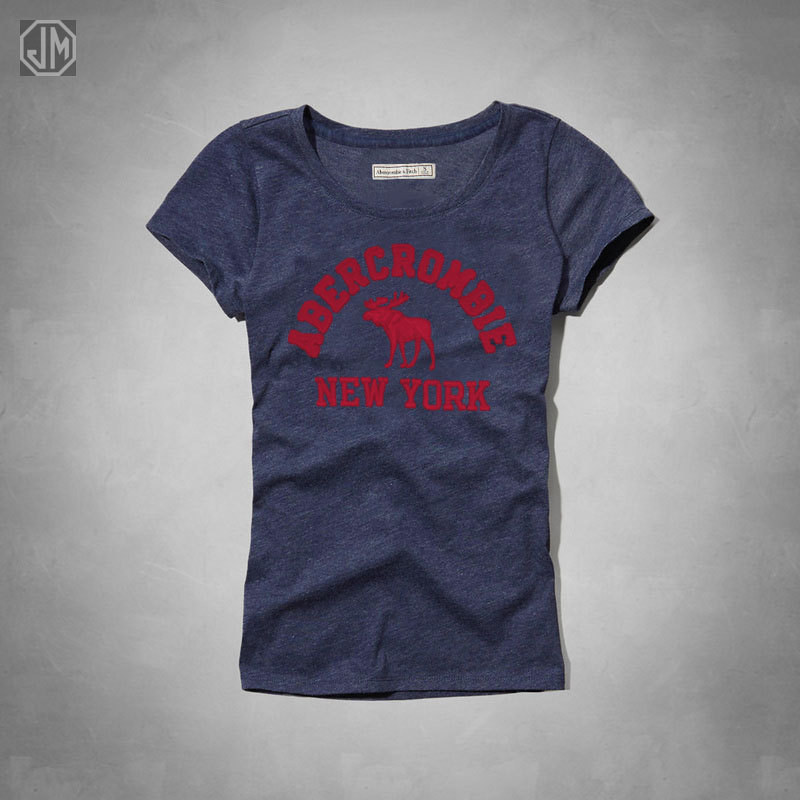The image features a blue t-shirt with a textured white and blue pattern, lying on a light gray background that is brighter in the center and darker in the corners. Positioned at the top of the image, there is an octagon with the letters "JM" inside it, outlined in light gray. Dominating the center, the t-shirt showcases a prominent red semicircle with bold text spelling out "Abercrombie" across the chest. Below the text, an outlined moose with horns is depicted walking to the left. Beneath this, in smaller dark red capital letters, is the text "New York." The shirt, which has short sleeves on either side, features some natural creases and folds. Inside the back collar, a white rectangular label can be seen, potentially bearing the brand name "Abercrombie & Fitch" in black.